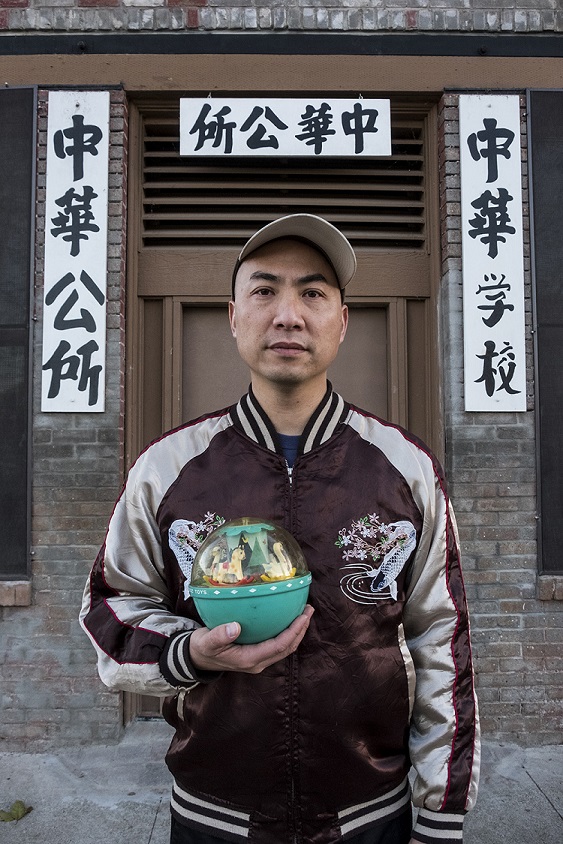The image features an Asian man standing in front of a brick building with a restaurant that has East Asian characters above the doorway and banners with additional kanji symbols hanging on each side. He is holding a green, globe-like object in his right hand, which appears to be a plastic dome covering a carousel-like diorama with figures of a horse and a swan inside. The man is wearing a maroon and white windbreaker-style jacket adorned with fish and sakura blossoms, detailed with blue fish and pink, green, and white flowers. He also wears a tan baseball cap. The man stands on a gloomy, somewhat dirty sidewalk, looking directly at the camera with a neutral expression, appearing disgruntled and maintaining a rather stiff posture.